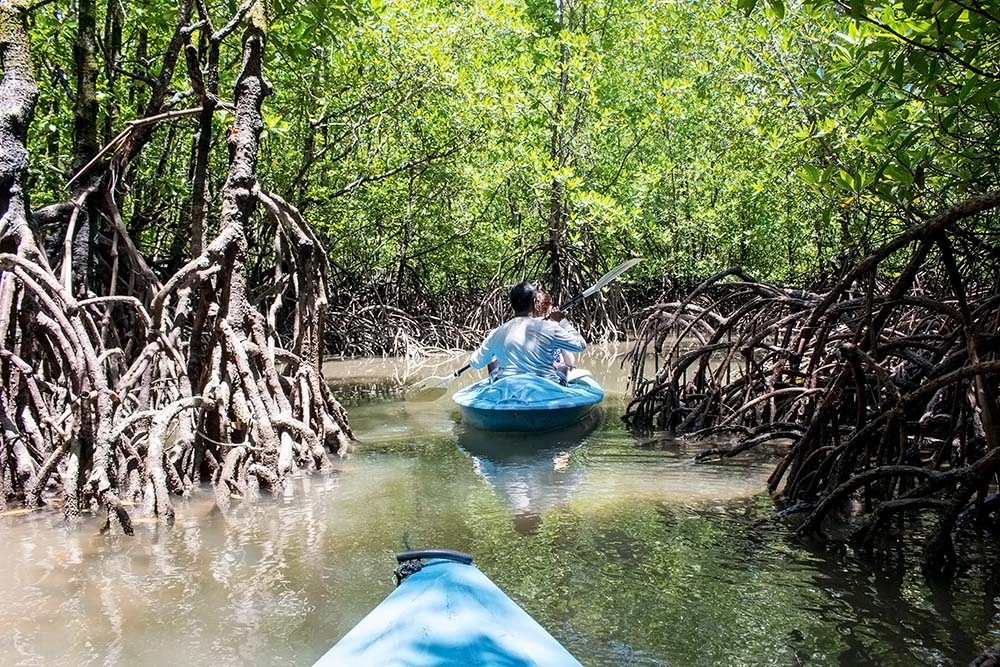This photograph captures an adventurous kayak trip through a swampy creek, surrounded by dense, intertwined tree branches and vibrant green foliage. In the foreground, the tip of a light blue kayak is visible, hinting that the photographer is also in a kayak. The murky brown water below reflects the unique root systems of the trees, which extend conspicuously above the surface. In the background, a man in a white shirt paddles another blue kayak through the winding, hedge-like groves. Sunlight filters through the canopy of leaves, creating a picturesque scene of illuminated greenery amid the swampy waters.